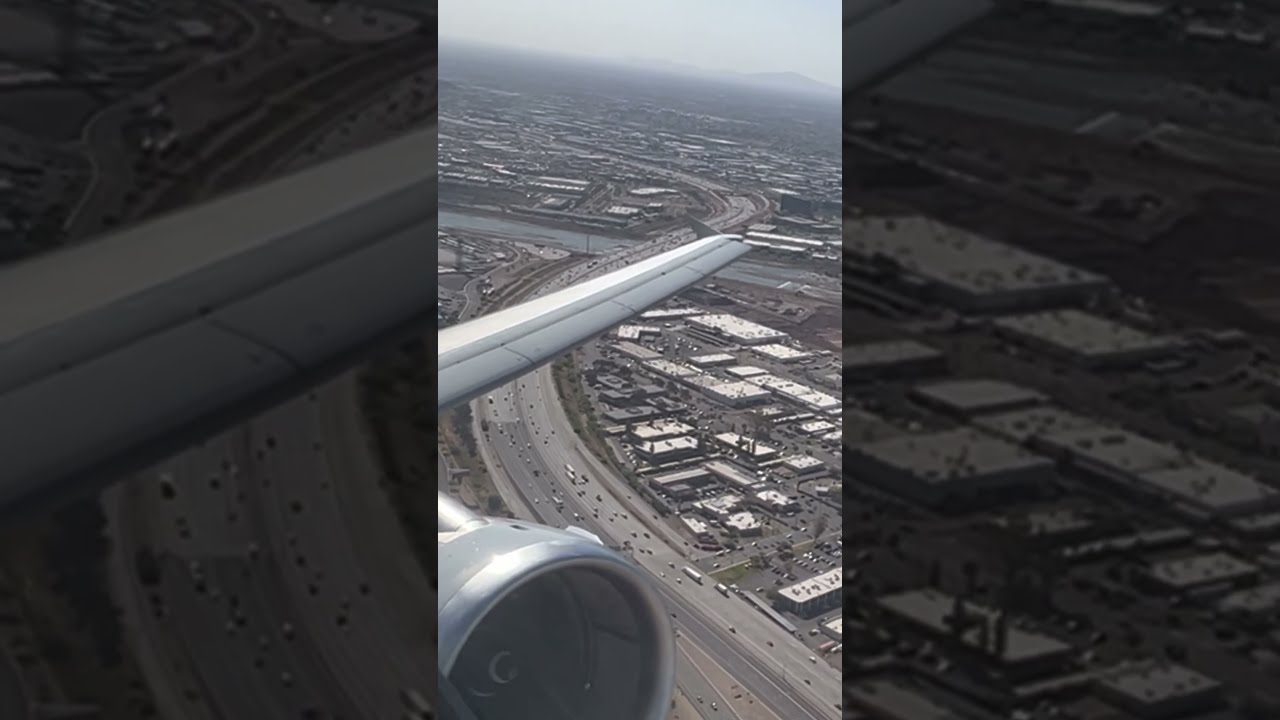This is a vertical, exterior daylight photograph of a cityscape taken from a plane window, most likely with a cell phone. The image, split into three sections with the outer ones being darker and monochromatic, comprises a central color photo that vividly captures the scene below. Dominating the foreground, the left side showcases the airplane's wing and jet engine, stretching across the image from left to right. Below, a sprawling, multi-lane highway—varying from four to eight lanes—meanders in a zigzag pattern. The road is modestly trafficked, weaving through a semi-dense city filled with low-lying buildings, likely industrial facilities with bright white roofs. A river with a bridge intersects this highway, adding to the complexity of the urban landscape. The horizon is hazy, possibly due to overcast skies, and there are faint suggestions of hills or mountains in the distance.